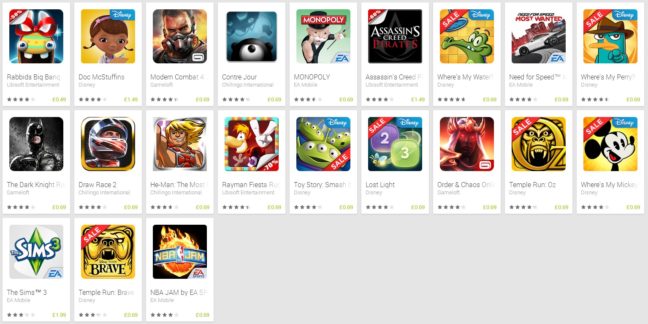The image features a grid layout showcasing 21 different apps, each represented on a small white card against a large gray background. Arranged in three rows, the first and second rows each contain 9 apps, while the third row has just 3. Each card includes a graphic representing the app, with the app's name, publisher, and a 5-star rating system displayed below the graphic. On the right side of each card, the installation price for the app is prominently displayed. This orderly arrangement allows for a clear and concise presentation of various apps available for installation.